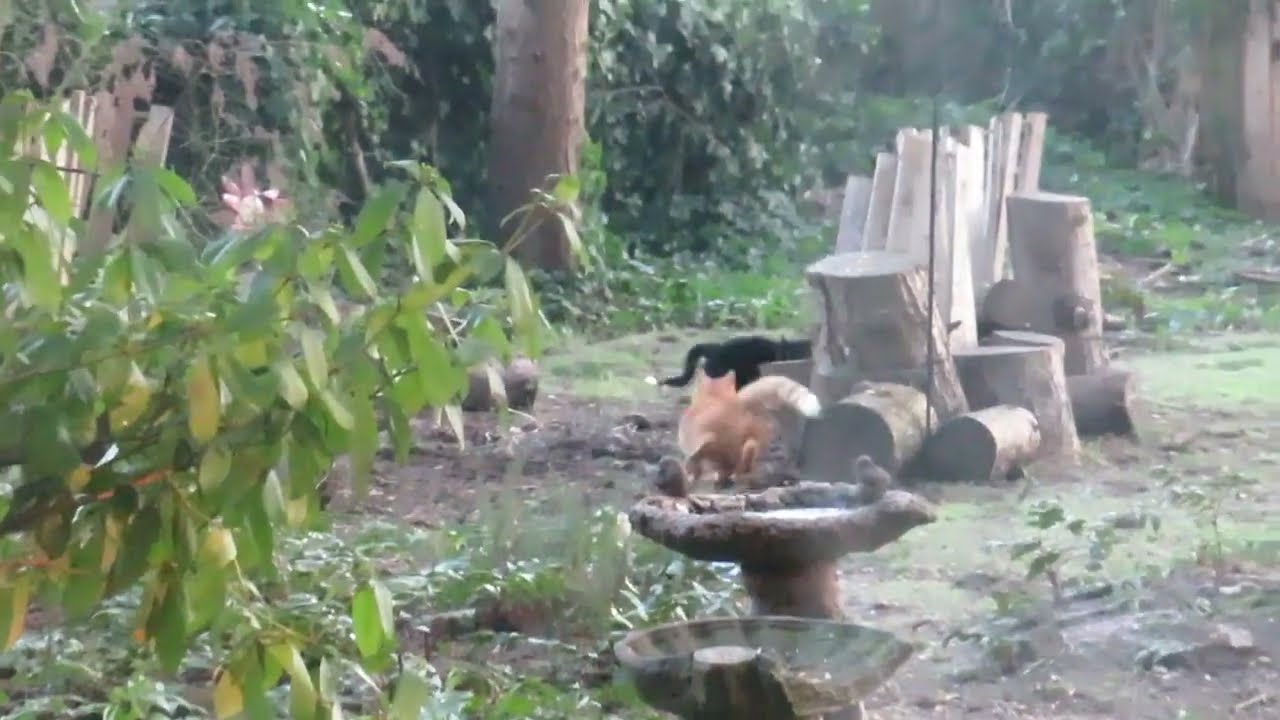The image depicts an outdoor, rustic scene with a slightly unusual, off-white hue. In the foreground, two weathered and irregularly shaped fountains or birdbaths can be seen, some of which seem to be in disrepair and one possibly hosting birds. On the left side, green leaves partially obstruct the view. In the midground, there appears to be a blurry brown cat, possibly accompanied by another, observing something indistinct and black that might also have a tail. Surrounding the animals are a number of tree trunks and sawed-off logs—some standing, others scattered on the ground. Stacked wood can also be seen, looking as if it has been partially chopped. Toward the background, dense greenery and several more tree trunks frame the scene, with patches of grass and exposed dirt visible on the ground. The entire image has a peculiar, almost monochromatic tint, making the wood appear white instead of its natural brown color, and the ground grayish. There are also some boards standing upright in the background, contributing to the sense of a somewhat cluttered and overgrown area.